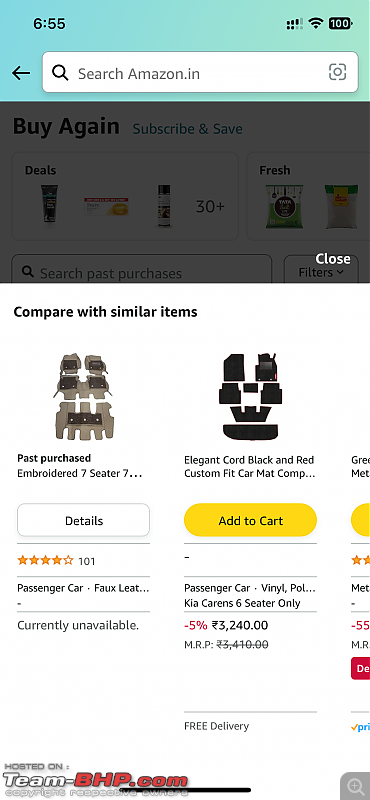The Amazon webpage being viewed showcases a variety of features and options available to the user. At the top of the page, there's a prominent search bar for easy navigation. Below this, a "Buy Again" option is accessible for users to repurchase previously bought items quickly. 

Currently, the focus is on the "Compare with similar items" section, highlighting seat covers. One of the featured products is an embroidered, beige 7-seater seat cover, though it is currently unavailable. This product has received a rating of 4 out of 5 stars based on 101 customer reviews. The seat cover is designed for passenger cars and is made of faux leather.

Another seat cover option presented is a black and red cord design, available in vinyl and polyester. Users can add this product to their cart, and it comes with the benefit of free delivery. Additionally, some information is listed in another language, possibly indicating international availability.

Adjacent to the seat covers, there's a section hosted on teambhp.com featuring similar items. Above these sections, there is a black dialog box that, when closed, reveals more options like the "Buy Again" section where users can subscribe and save on repeated purchases. This section highlights various deals, including items such as toothpaste and other products in tubes. There are over 30 items listed for convenient reorder. 

Lastly, the page features an "Amazon Fresh" section, which offers users the ability to purchase produce and other perishable grocery items directly from Amazon.